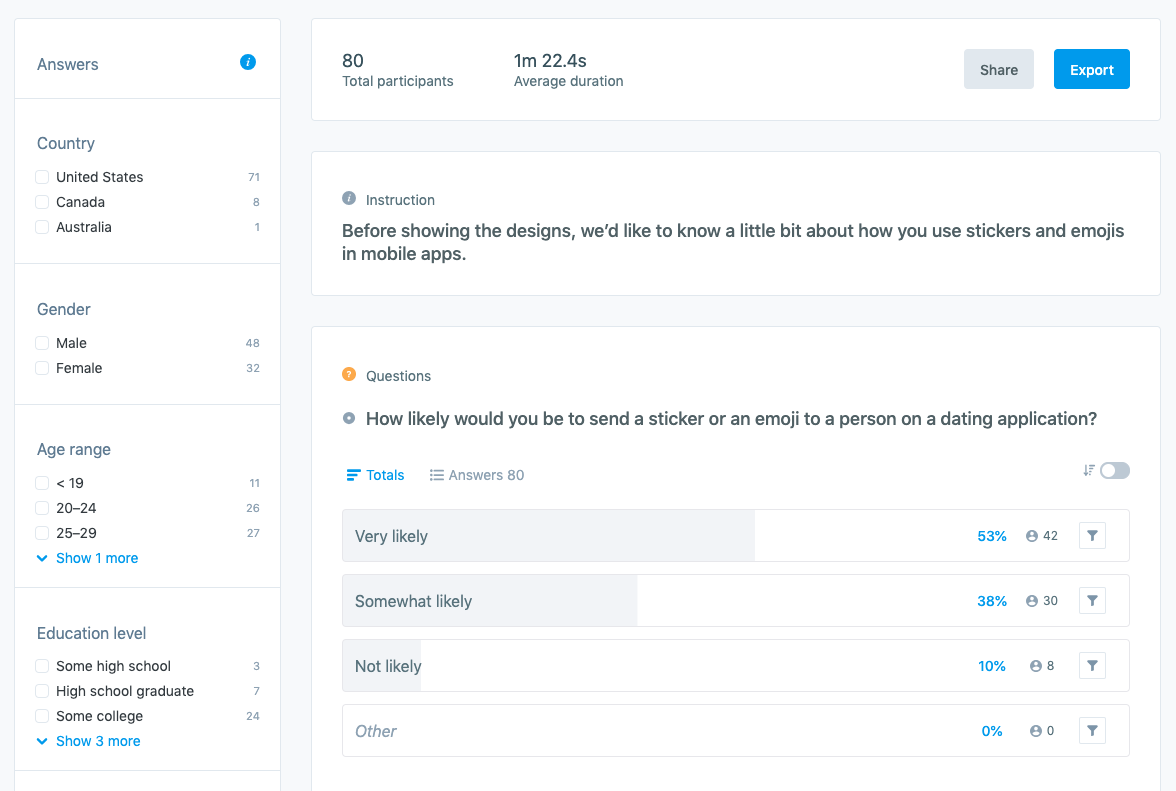The screenshot appears to be from a metrics dashboard focusing on user demographics and survey responses. On the left side, there's a filtering menu allowing for various customization options. These filters include categories like 'Country' with checkboxes for the United States, Canada, and Australia; 'Gender' with options for Male and Female; 'Age Range' segmented into less than 19, 20 to 24, and 25 to 29 with an option to "show more"; and 'Education Level' with options such as some high school, high school graduate, and some college along with a "show more" option.

On the right side of the screen, a summary box at the top displays key metrics: "80 total participants," "1 minute, 22.4 seconds average duration," and features for sharing and exporting data with a blue 'Export' button. Below these metrics, an instruction box provides context: "Before showing the designs, we'd like to know a little bit about how you use stickers and emojis in mobile apps."

Further down, in a separate 'Questions' box, a specific survey question is presented: "How likely would you be to send a sticker or an emoji to a person on a dating application?" Response options are detailed with their respective percentages: 'Very likely' at 53%, 'Somewhat likely' at 38%, 'Not likely' at 10%, and 'Other' at 0%.